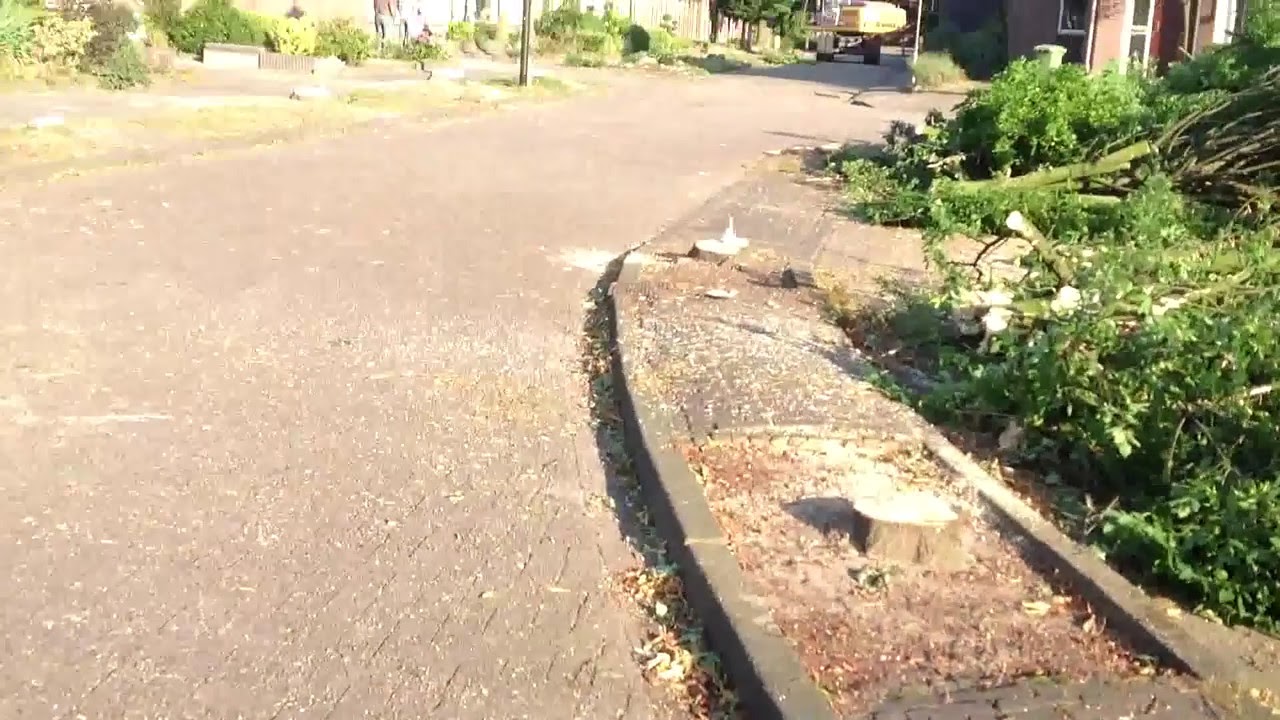This daytime photograph captures a detailed and vivid scene of a road and its surroundings. The grey road, lightly scattered with dry leaves and flower petals, starts at the bottom of the image, stretching upwards towards the center where it splits off — curving to the right and branching straight ahead. On the right side of the road, a raised concrete footpath features two tree stumps with roots still in the ground, indicating that the trees have been recently cut. The green leaves and branches of these felled trees are piled up alongside the footpath. Beyond the footpath, there are freshly cut plants with green leaves and severed stems. On the left side of the road, intact green plants flourish. Further away, lining both sides of the street, are a few buildings. At the top center of the photograph, a large vehicle is visible, moving away from the viewer. The colors in the photograph include shades of grey, green, tan, brown, white, and yellow, contributing to the vibrant, outdoor setting in what appears to be a small town bathed in bright daylight.